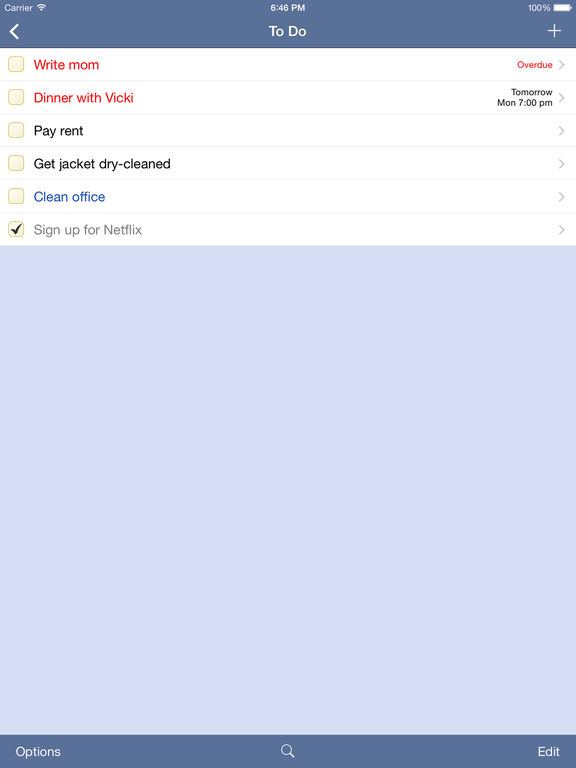This image is a detailed screenshot of a to-do list displayed on a person's cell phone. At the top of the screen, a dark grayish-blue banner is visible. On the top left, the banner displays the word "Carrier," followed by the Wi-Fi icon. The time "6:46 PM" is centered in the banner, while the battery icon, indicating a 100% charge, is positioned on the right.

Below the banner, the interface features a navigation arrow pointing to the left, the title "To Do" in white letters, and a white plus sign, all on a white background. The to-do list items are organized sequentially, each separated by a thin gray horizontal line. The list includes the following items:

1. "Write Mom" marked as "Overdue."
2. "Dinner with Vicki," scheduled for "Tomorrow, Monday, 7 PM."
3. "Pay Rent."
4. "Get Jacket Dry Cleaned."
5. "Clean Office."
6. "Sign Up for Netflix," which has been checked off as completed.

The bottom portion of the image transitions to a light gray color background. At the very bottom, a dark grayish-blue section displays three options in white letters: "Options," a magnifying glass icon for "Search," and the word "Edit," located at the bottom right corner. The format of the image is portrait-oriented, revealing no photographic elements, and it does not feature any people, animals, plants, flowers, or trees.